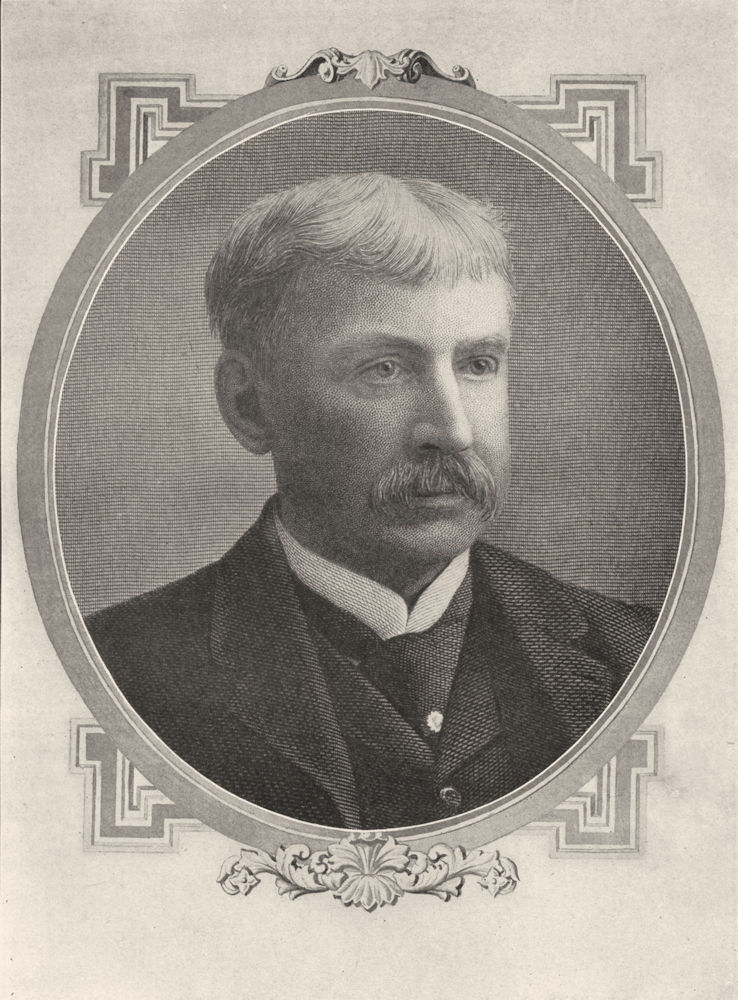The image depicts an elderly man from a different time period, likely several hundred years ago, captured in a black and white photograph. This man, who appears to be in his mid-middle age, has a distinct short hairstyle and a bushy mustache. He is dressed in a formal, multi-layered suit, which includes a vest, a necktie, and a white collared shirt, all contributing to his dignified appearance. The entire photograph is meticulously centered, with the man positioned perfectly at the heart of a circular portrait frame. This frame, decorated with artistic embellishments and geometric designs at the top and bottom, draws further attention to the man at its center. The simplicity of black, white, and grey tones adds an old-world charm, emphasizing the vintage nature of this image.